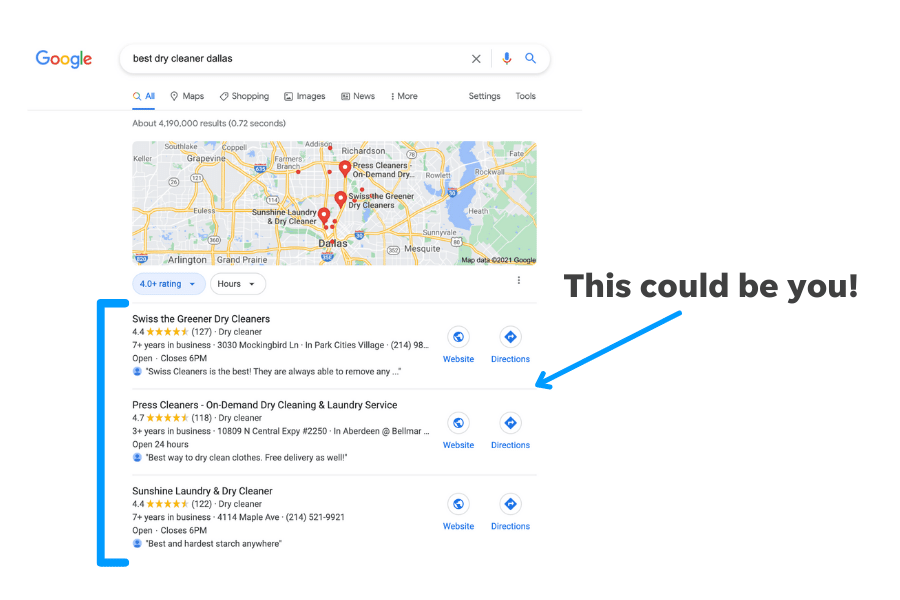Image Description: The screenshot captures a Google search results page. Dominating the upper left corner is the iconic Google logo. Below it spans the search bar, which contains the typed query "best dry cleaner Dallas" in lowercase. To the right of the search bar, there are several icons: an 'X' for clearing the search, a microphone for voice input, and a blue magnifying glass to initiate the search.

Immediately below the search bar, the navigation menu offers various categories: "All," "Maps," "Shopping," "Images," "News," along with "More," "Settings," and "Tools" options. Beneath this menu, it shows search results information: approximately 4,190,000 results, which were found in 0.72 seconds.

The main body of the page displays a Google Map featuring three red location markers indicating dry cleaner locations in Dallas. Below the map, the search results are detailed. 

1. **Swiss the Green Dry Cleaners**: The first result, with its name highlighted, followed by star ratings, a brief description indicating its 7+ years in business, its address, phone number, and operating hours.

2. **Press Cleaners - On-Demand Dry Cleaning and Laundry Service**: The second result, presenting a similar layout, indicates a 4.7-star rating and details its 3 years of service, address, and other essential information. A subtle blue arrow points to this entry suggesting further relevance.

3. **Laundry and Dry Cleaner**: The third entry, with minimal details except its Texas location, potentially indicating a new or less known business.